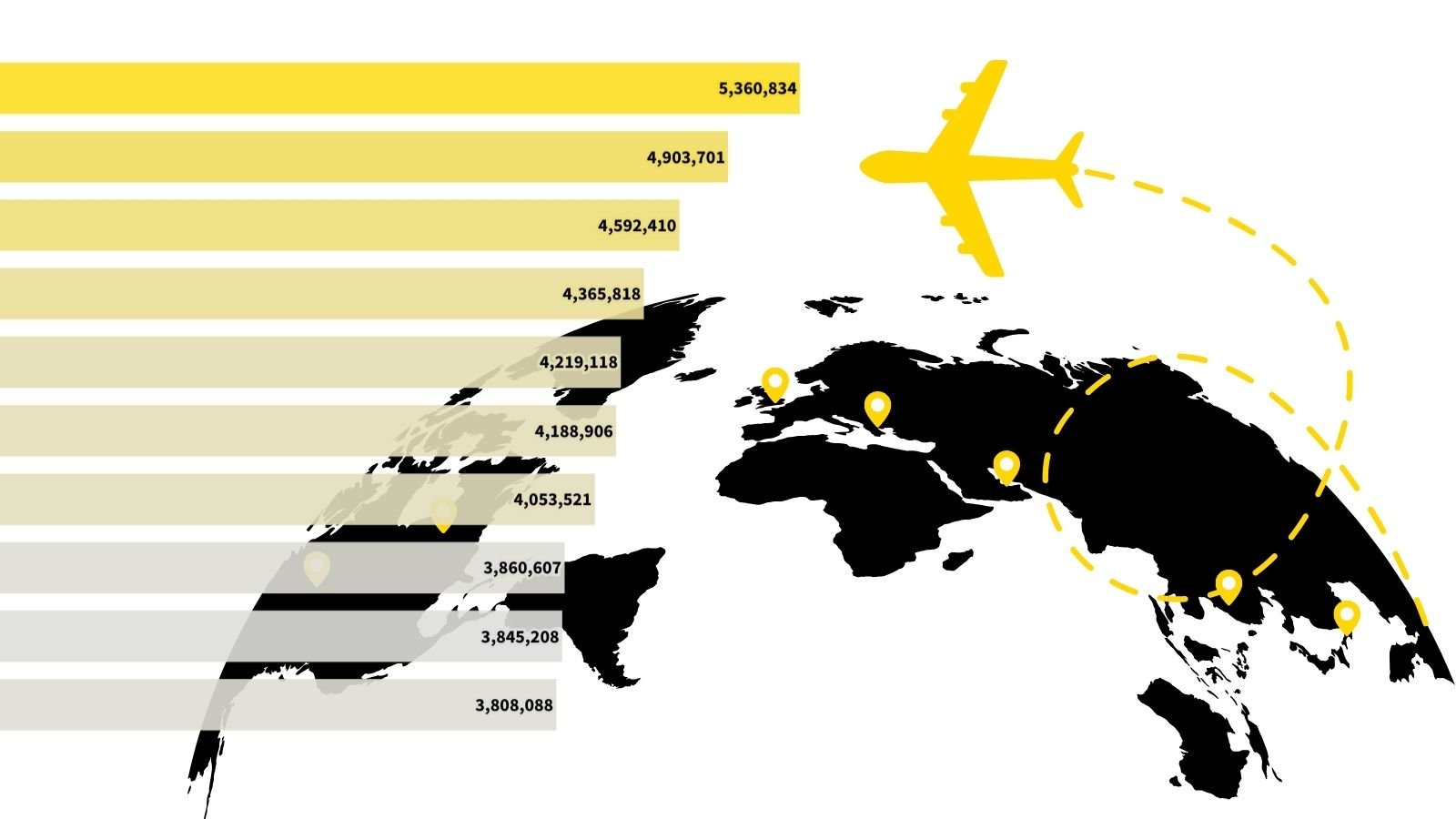This is a detailed illustrative graphic presented in a crisp, clear, high-quality format. Dominating the image is a black and white globe that showcases slightly more than half of its surface. Black continents are accentuated with gold pop-up bubbles, each containing a white circle. Above the globe, gold dashed lines intersect the sky, leading a golden airplane flying overhead. On the right side of the image, an array of gold bars is displayed, marked with black numbers. The bars transition from gray at the bottom to gold at the top, creating a gradient effect. The image is minimalistic with no additional objects, ensuring a clean and focused presentation.